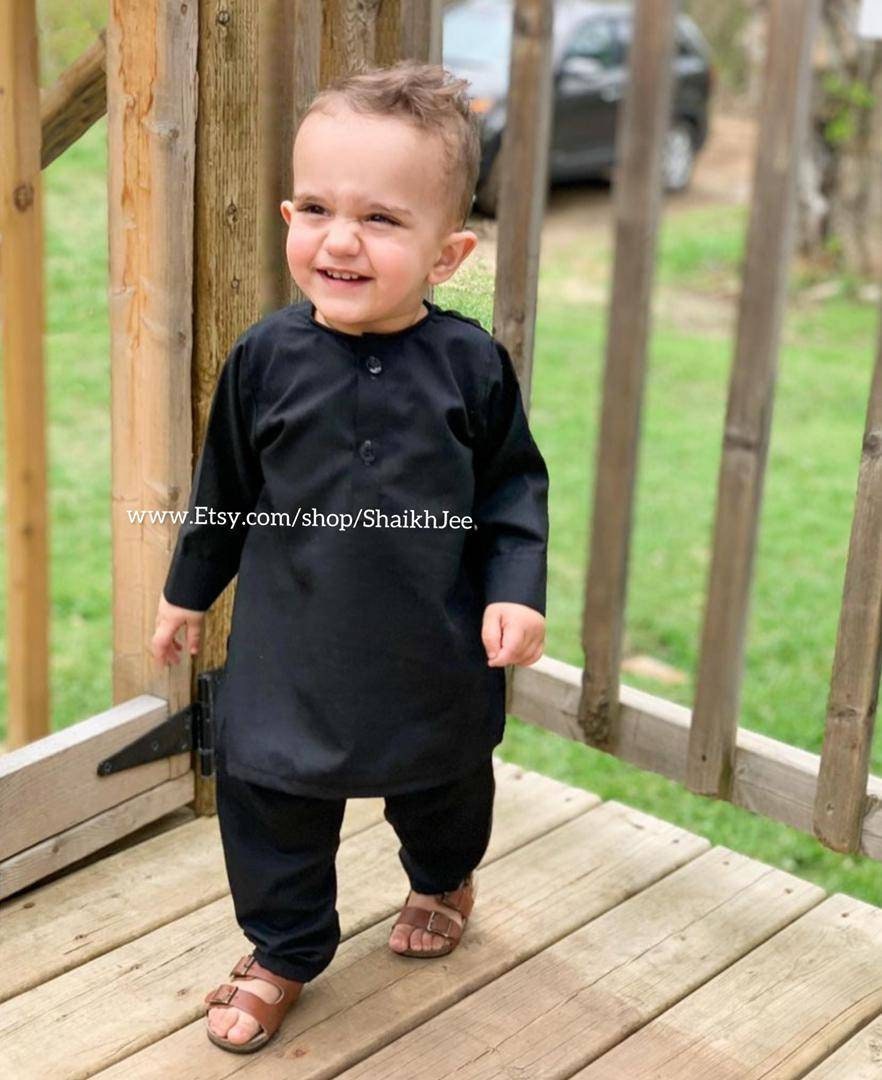The photograph depicts a young, white toddler dressed in traditional Muslim attire, composed of a black tunic top with long sleeves that extend past his waist, black pants, and brown sandals with two buckle straps. His tunic features either two or three buttons on the chest. The boy has messy hair, slightly pointy ears, rosy cheeks, and an expressive face that appears to be scrunched up in a smile, showcasing his little teeth. He stands on a light brown wooden deck, which seems to be part of a porch area, with a wooden railing and gate visible behind him. In the background, there's a driveway with a gray SUV. The overall scene is outdoor, taken during the day, and part of the photograph includes text promoting an Etsy shop: www.etsy.com/shop/shaikhjee.